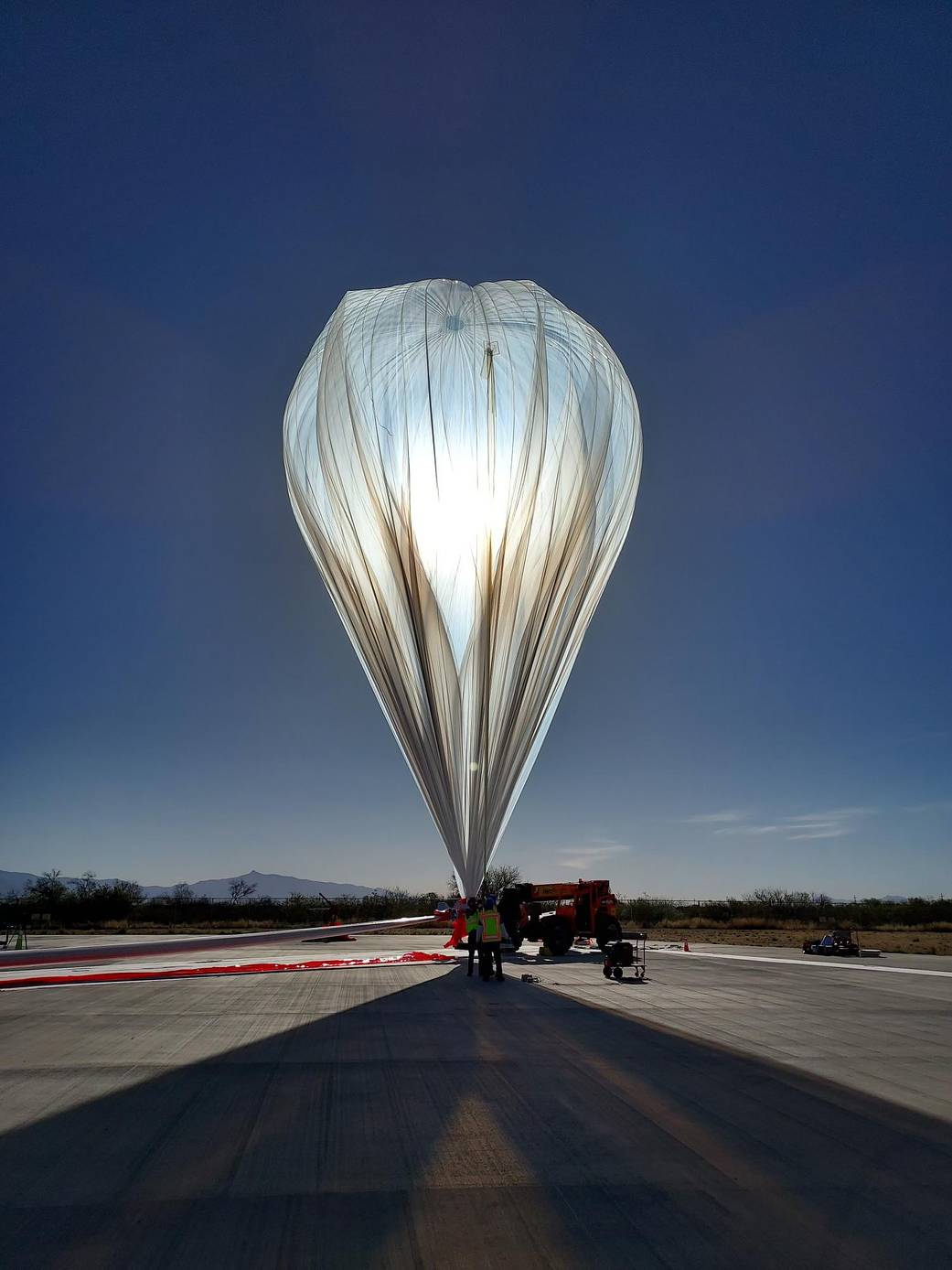In this vertically aligned outdoor photograph, the central focus is a large, inverted teardrop-shaped weather balloon made of white and brown cloth. The balloon is anchored on what appears to be a runway, with a bright white light radiating from its center, casting a significant triangular shadow downward. The background features a dark blue sky transitioning to a lighter blue with wispy white clouds as it nears the horizon, suggesting the time of early morning or early evening. 

Nearby the balloon, a gray truck and a small cart are parked to the right, with a couple of people standing at the balloon’s base, indicating the scale and providing a sense of activity. The lower portion of the image is dominated by a road leading towards the balloon, converging at a single point. A long red and white banner lies on the ground to the left, while the backdrop includes a hint of flat terrain with a distant, low-lying elevation, possibly a hill or small mountain. The sky occupies most of the upper part of the image, contributing to the serene and expansive atmosphere. The intense brightness at the balloon's center suggests the sun might be positioned directly behind it, shining through the material and making it glow vividly.